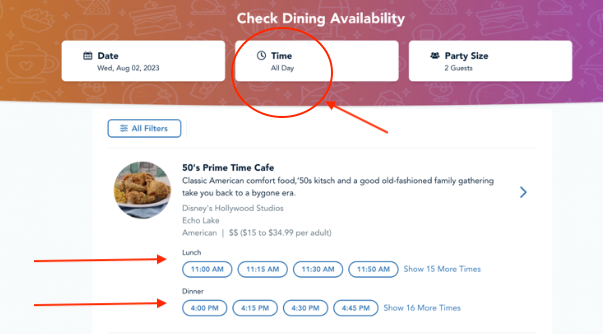In this screenshot of a restaurant reservations page, the top section is dominated by a vibrant, colored rectangular header that transitions from orange to purple, adorned with faint white illustrations of various food items. At the top in white text, the header reads, "Check Dining Availability." Beneath this header, three rectangular selection boxes are displayed horizontally.

The first box is labeled "Date," displaying "Wednesday, August 2, 2023." The second box is labeled "Time," showing the parameter "All Day" in gray text. The third box on the right is labeled "Party Size," indicating "2 Guests" in gray text.

Below the header, against a white background, lies a blue rectangular button labeled "All Filters." This is followed by the first restaurant entry. Titled "50's Prime Time Cafe," this section includes a brief description of the cafe's atmosphere and type of food, accompanied by a circular image of a plate of fried chicken. Below the description, the location is specified in gray text as "Disney's Hollywood Studios, Echo Lake," and the type of cuisine is listed as "American."

The restaurant section also includes a price range indicator. Below this information are two rows showing available reservation times. The first row, for lunch, offers time slots such as 11:00 AM, 11:15 AM, 11:30 AM, and 11:50 AM, with an option to "Show 15 More Times," indicated by a red arrow. The second row, for dinner, lists times starting from 4:00 PM, followed by 4:15 PM, 4:30 PM, and 4:45 PM, with an option to "Show 16 More Times," also marked by a red arrow.